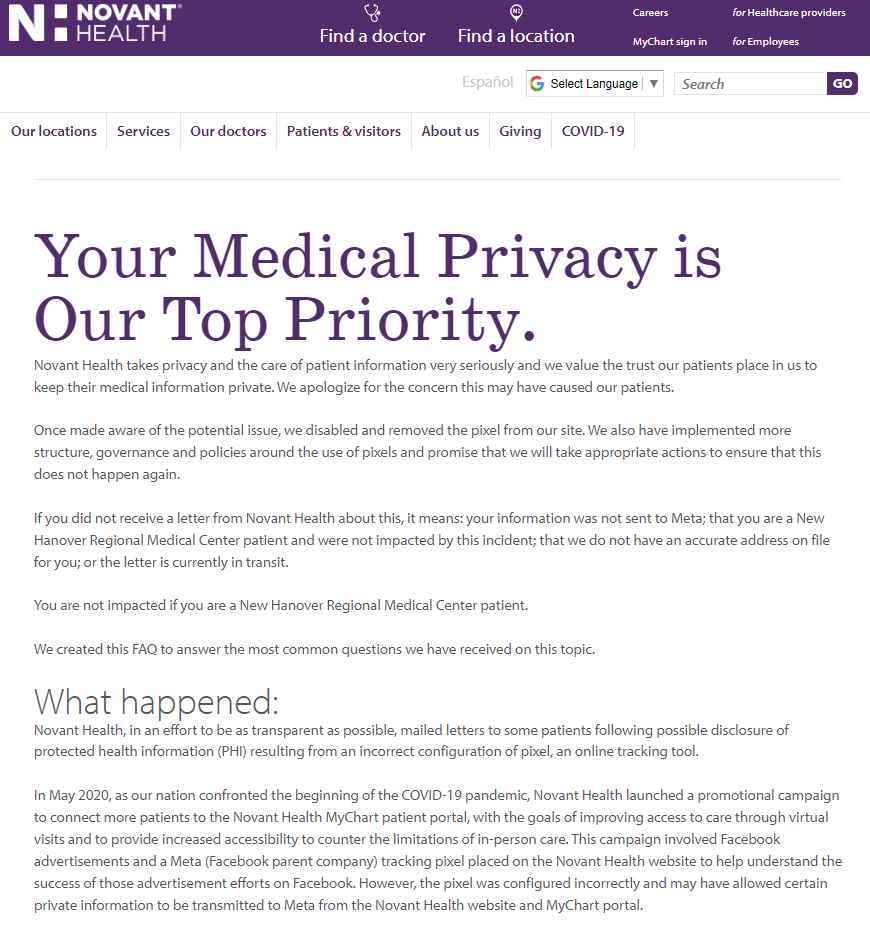The webpage on the Novant Health website is thoughtfully designed for easy navigation and user convenience. At the top, there are primary tabs for essential features: "Find a Doctor," "Find a Location," "Careers," "My Chart," "Sign In," a section for Healthcare Providers, and another for Employees. Just below these tabs is a Google Translate drop-down menu and a search box, facilitating multilingual access and quick searches.

The main navigation bar provides links to critical sections, including "Our Locations," "Services," "Our Doctors," "Patients & Visitors," "About Us," "Giving," and "COVID-19." 

An article prominently featured on the page emphasizes the importance of medical privacy, titled "Your Medical Privacy is Our Top Priority." Following this title is detailed text elaborating on their commitment to patient confidentiality. Below this, another paragraph addresses "What Happened," likely providing further information or context to the main article.

Overall, the Novant Health website ensures users can efficiently find the information they need, from healthcare services and doctor locations to career opportunities and patient privacy information.